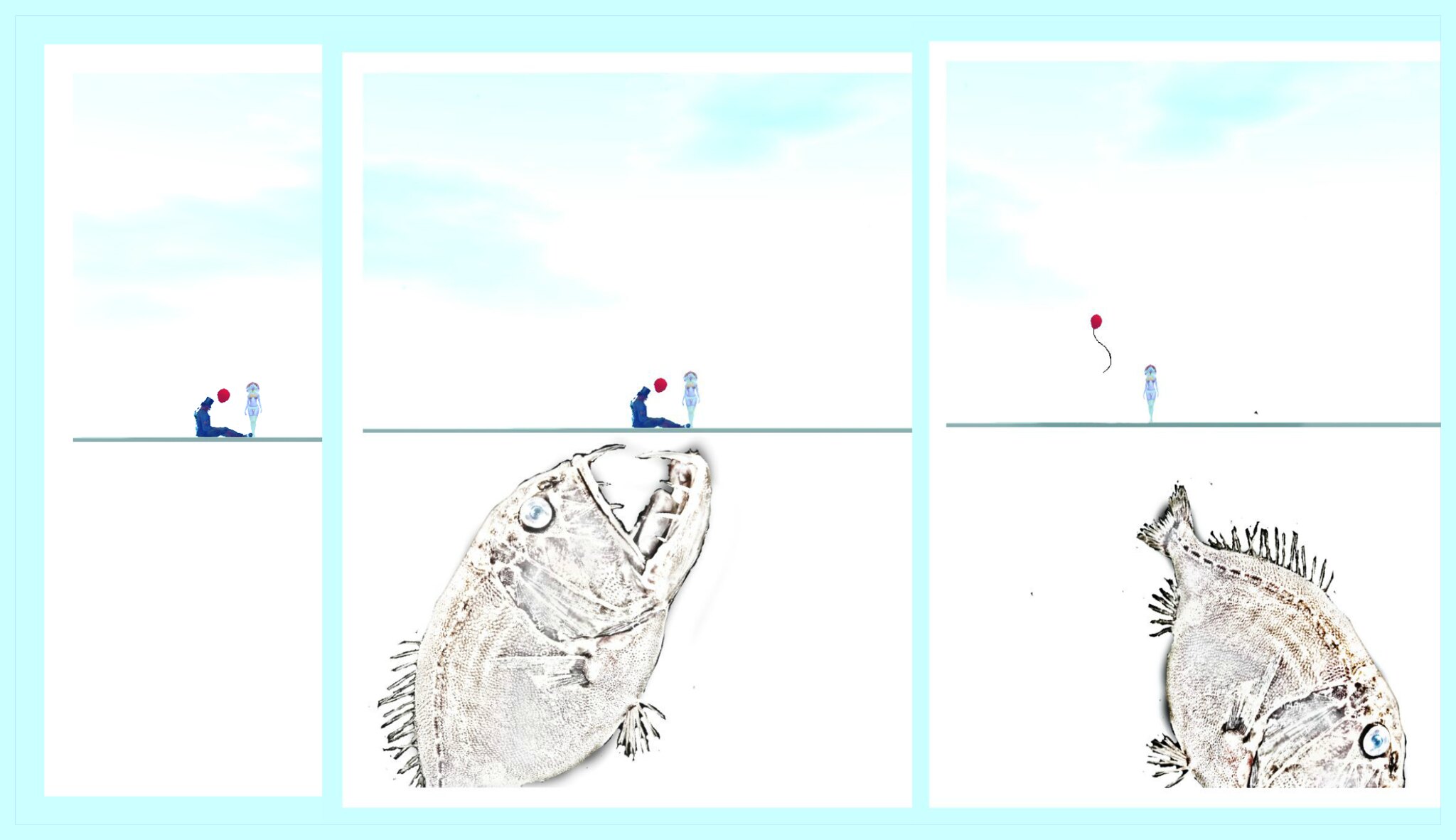This is a detailed watercolor painting composed of three vertically oriented sheets of paper, arranged in a sequence on a bright turquoise surface. Each paper has slightly different dimensions but together form a continuous horizontal scene. At the top half of each sheet, a pale blue and white sky with subtle blotches creates an impression of a cloudy atmosphere. A horizontal green line runs across the center, representing the ground. 

The scene features two silhouettes: an adult sitting in profile, rendered in dark blue, facing right, and a child in a lighter blue, standing and facing forward. The adult figure is depicted holding a red balloon near their head. In the middle and right sheets, a large, menacing anglerfish with sharp teeth and cloudy eyes dominates the lower half. In the middle section, the fish's mouth is open wide as it seemingly targets the adult figure. By the third sheet, the adult has vanished, implying they have been consumed, and the fish is seen diving away with its tail visible. The red balloon floats upwards, now left alone with the child silhouette on the ground.

The entire artwork is marked by strong contrasts, with the bright turquoise background making the whites appear starkly blown out, enhancing the dramatic visual narrative.